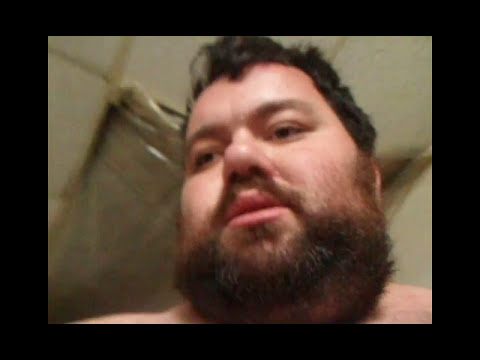This photograph features a close-up of a man's face framed within a thick, black rectangular border. The man's face and shoulders occupy the top right portion of the image. He has short, cropped brown hair, a full and sizable brown beard, and brown eyes. The lighting and quality suggest a low-resolution selfie, possibly taken from a slightly below angle. The man appears to have a neutral, blank expression and is gazing off to the left. The background behind him seems to be a bathroom with white tiles and a towel rack, though some descriptions suggest a more ambiguous setting with white panels or tiles. The image itself measures approximately 5 inches wide by 4 inches tall and does not feature any additional text or images. The man is not wearing a shirt, adding to the possibility that he is in a bathroom setting.